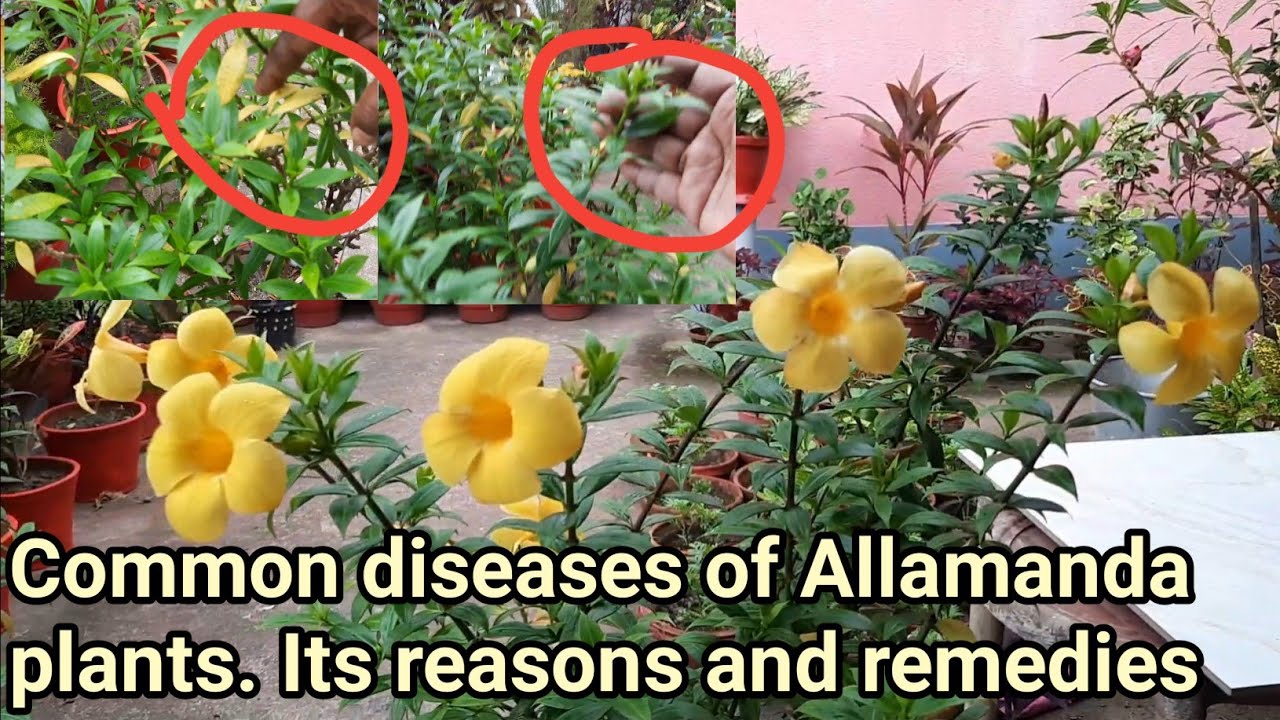The image features a detailed display of common diseases affecting Alamanda plants, along with their causes and suggested remedies. At the bottom of the photo, bold yellow text outlined in black reads, "Common Diseases of Alamanda Plants, Its Reasons and Remedies." The image showcases a variety of Alamanda plants with long green stalks and vibrant yellow flowers, set against a pink and blue background that suggests a nursery or greenhouse setting filled with numerous potted plants. 

In the top left, a hand is pointing to a discolored leaf, which has turned yellow and has been circled in red marker to highlight the issue. Another hand in the top right is cupping a leaf that appears dull and less vibrant, also circled in red marker. Some of the surrounding leaves are a healthy green, while others show signs of distress with tinges of red. The image effectively uses hands and red markings to draw attention to the specific issues with the plants, emphasizing the visual symptoms of the diseases being discussed.